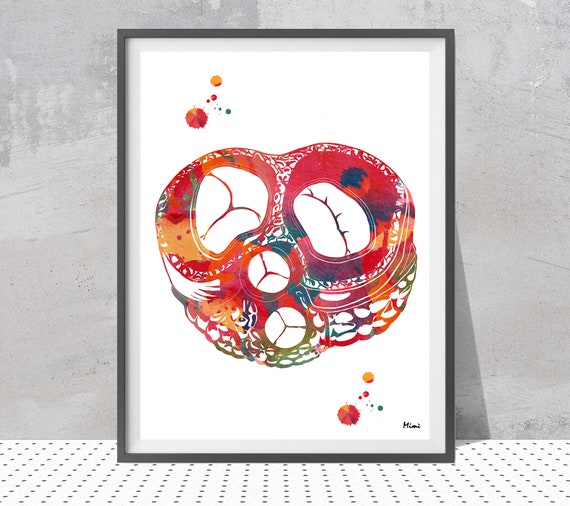This photograph captures a framed abstract print, leaning against a very light gray stucco wall. The print appears to be created with a printing press, showcasing a vibrant, multicolored design comprising shades of red, blue, green, orange, pink, and purple. It is held within a black frame and features a white background. The abstract design is characterized by amorphous, blob-like shapes interspersed with irregular, circular openings. Tiny splatters of color adorn the top right and lower right corners of the piece, adding a dynamic feel. The surface beneath the frame is white, covered in small black dots, resembling either a cloth or a countertop. The artist’s signature, "Mimi," is visibly inscribed at the bottom of the artwork. The frame casts a shadow on the wall behind, enhancing the depth and texture of the overall composition.